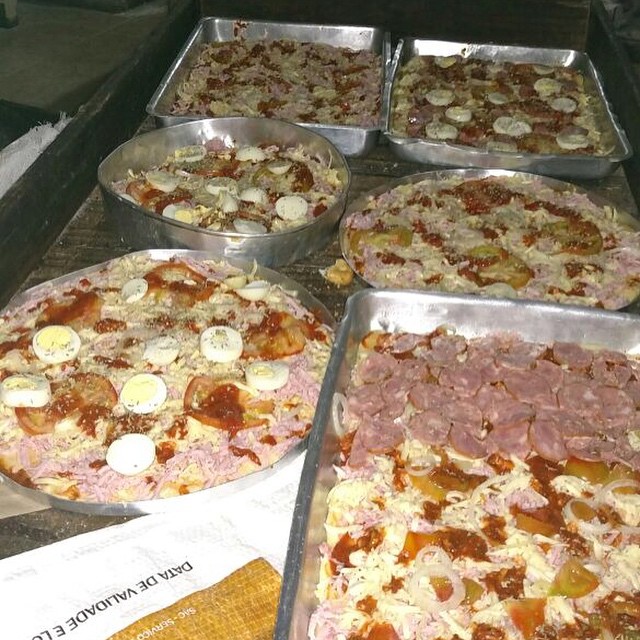The photograph showcases an assortment of six homemade pizzas, arranged along a covered table. The pizzas are presented in an eclectic mix of pans, ranging from rectangular and square baking pans typically used for cakes, to round shallow and tall pans that might traditionally be used for pies or cakes. Each pizza features unique toppings but shares common elements, such as sliced hard-boiled eggs and a pinkish shredded cheese. 

The pizza nearest to the bottom left corner is nestled in a rectangular pan and piled with slices of what looks like pepperoni, red sauce, cheese, and onions. Adjacent to it, in a round, shallow pan, is another pizza adorned with hard-boiled eggs, red sauce, tomatoes, and the mysterious pink shredded cheese.

In the middle row, there are two more pans. On the left is a tall round pan with a pizza that has a chunk of garlic in the center, hard-boiled eggs, red sauce, and cheese. On the right, a pizza in a square pan carries the same motif of red sauce, cheese, and hard-boiled eggs.

At the top, the last row displays two square pans, each housing a pizza similar to the ones before them, with red sauce, cheese, and the unmissable hard-boiled eggs. Behind these rows of pizzas, a white document with mustard yellow print peeks in from the lower-left corner, possibly listing ingredients or preparation details. The scene appears dimly lit, suggesting it might be taken in a cooler.

Additionally, a bag on the table bears the text "Data de Validade," indicating some connection to Portuguese or Spanish, possibly referring to an expiration date. This diverse setup seems like a labor of love for a special event or gathering, characterized by its homemade touch and varied baking containers.